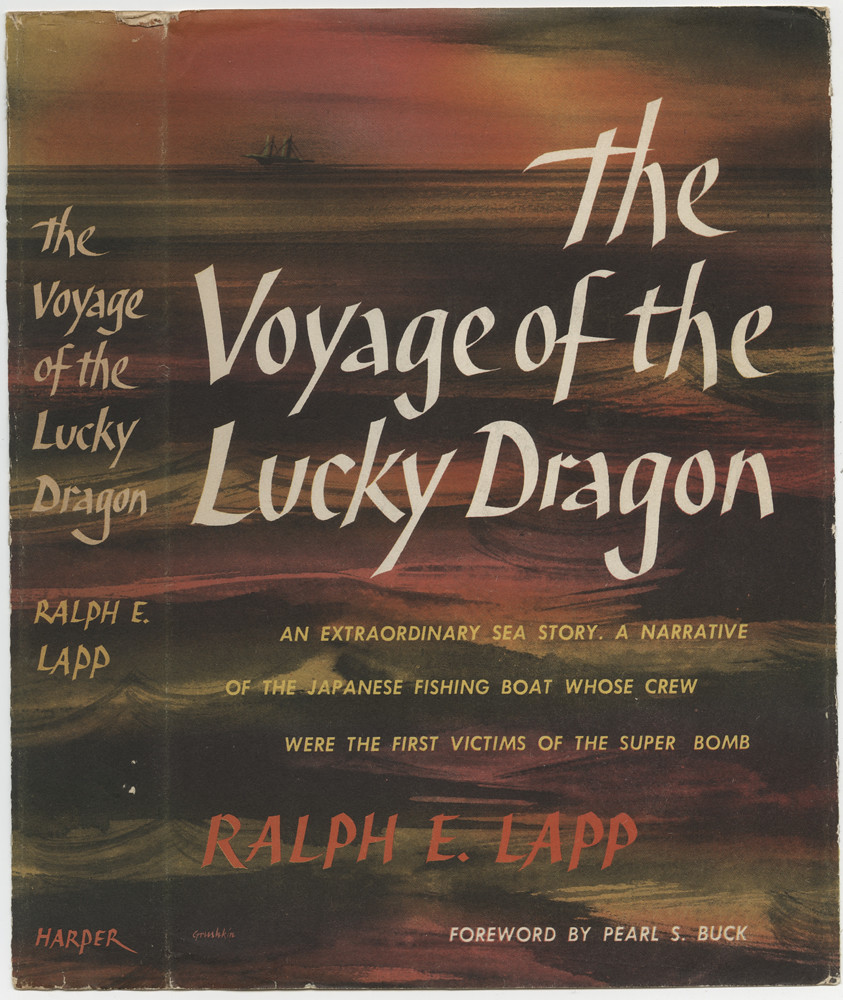The image depicts the flattened dust jacket of a book titled "The Voyage of the Lucky Dragon" by Ralph E. Lapp, with a forward by Pearl S. Buck. The cover features the book's title in white, with the subtitle "An Extraordinary Sea Story: A Narrative of the Japanese Fishing Boat Whose Crew Were the First Victims of the Superbomb" written in a smaller yellow font underneath. The author's name, Ralph E. Lapp, appears in red, and "Forward by Pearl S. Buck" is noted at the bottom right. The spine on the left repeats the title, author, and the publisher's name, Harper. The cover art showcases a painterly depiction of the sea, with predominant colors of reddish-orange and black, indicative of a sunset. The water covers about 80% of the background, reflecting the orange sunlight. On the horizon, there's a small double-masted ship amidst the waves, with clouds and an orangey sky filling the upper half. The entire design gives an impression of an old, weathered parchment with illustrations of ocean waves in black and dark green colors.